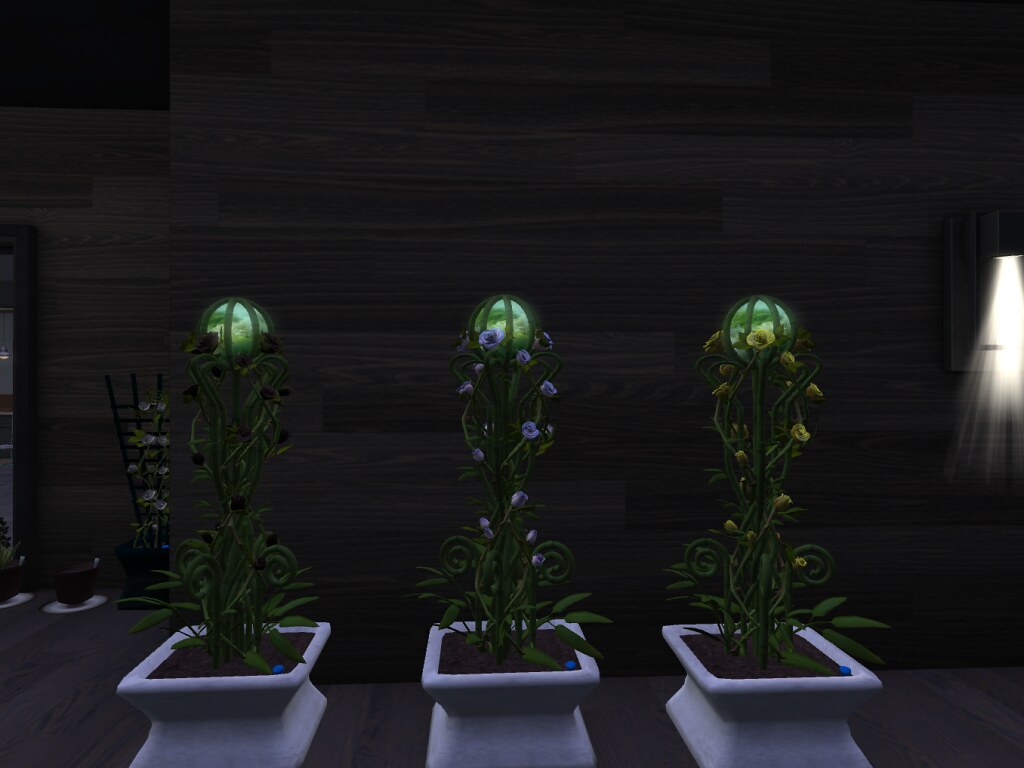The image presents a dimly lit, digitally-rendered scene inside what appears to be a wood-paneled room or cabin. Central to the composition are three distinct, white, square-shaped ceramic pots, each containing a tall plant. These pots feature a unique design with a bottleneck in the center, separating a top and bottom portion of equal dimensions.

Each plant possesses a swirling arrangement of leaves and displays flowers in different shades: the one on the left exhibits purple to dark blue flowers, the middle plant has lavender blooms, and the rightmost plant features yellow flowers. All three plants seem to spiral around a central pillar capped with a glowing, bright green orb that imparts a magical, fantasy-like ambiance to the scene.

The room features a wooden floor in a brown to grayish-brown hue and horizontal wood paneling on the walls. Additional elements include a sconce-type light fixture on the right wall and possibly a bookcase or TV to the left. In the background, there are also three more plant pots: a blue one with plants climbing a trellis and two smaller, reddish pots. The overall composition emphasizes the mystical feel, accentuated by the glowing orb and dim lighting, contributing to a serene yet enchanted atmosphere.